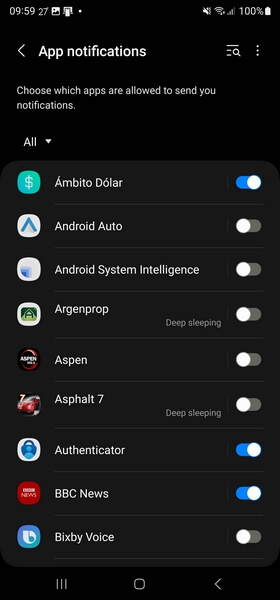This is a detailed screenshot of a phone's app notification settings page, likely from an Android device. The device's status bar is visible at the top, displaying essential indicators such as the time, battery level with a percentage, WiFi signal, and volume controls, confirming that this is from a mobile phone. The navigation bar at the bottom further supports this identification.

The notification settings page is titled "Choose which apps are allowed to send you notifications," and it presents a list of apps with their respective notification statuses. Some app names appear in English, including Bixby Voice, BBC News, Authenticator, Asphalt 7, and Android System Intelligence, while others are in what appears to be Spanish. The display reveals that certain apps are marked with a "deep sleeping" label, indicating they are in a low power state, and some apps have notifications enabled while others are disabled.

The phone's user interface is set to dark mode, with a black background designed to reduce eye strain and enhance readability in low-light conditions.